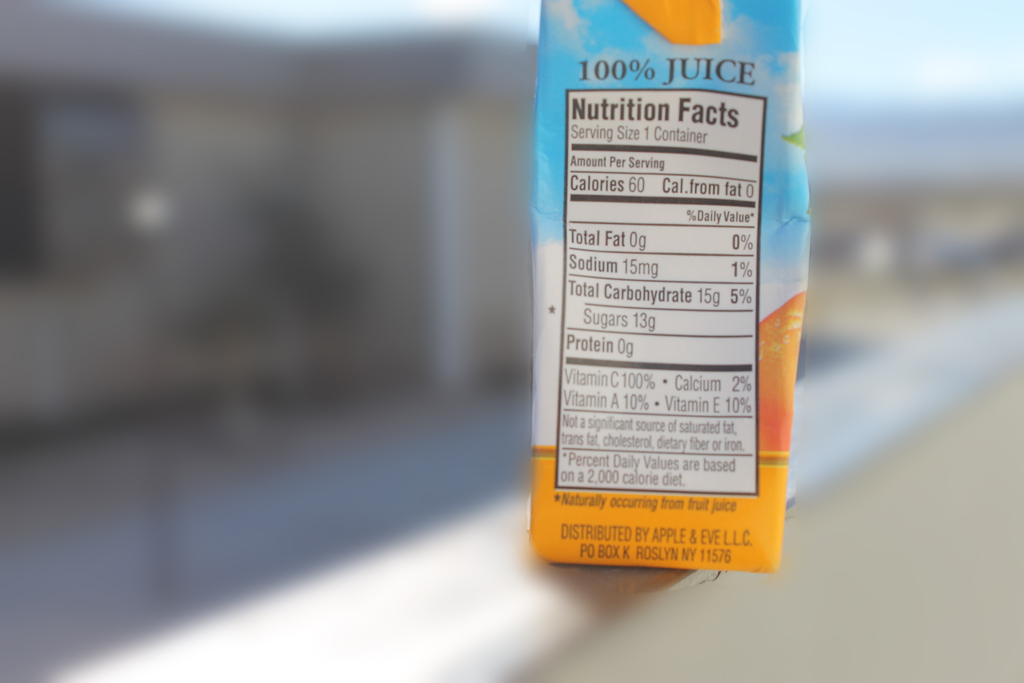The image features a vibrant carton of orange juice prominently placed on a raised surface, such as a wall. The carton, presented in sharp focus, boasts a vivid orange and blue design with a white panel displaying the nutritional facts. The detailed text reveals the juice is 100% pure, specifying the serving size as one container, along with caloric values and ingredient information. In the background, a single-storey white house can be perceived, although it remains deliberately blurred to accentuate the orange juice carton. The carton is distributed by Apple & Eve LLC, P.O. Box K, Roslyn, New York, 11576.